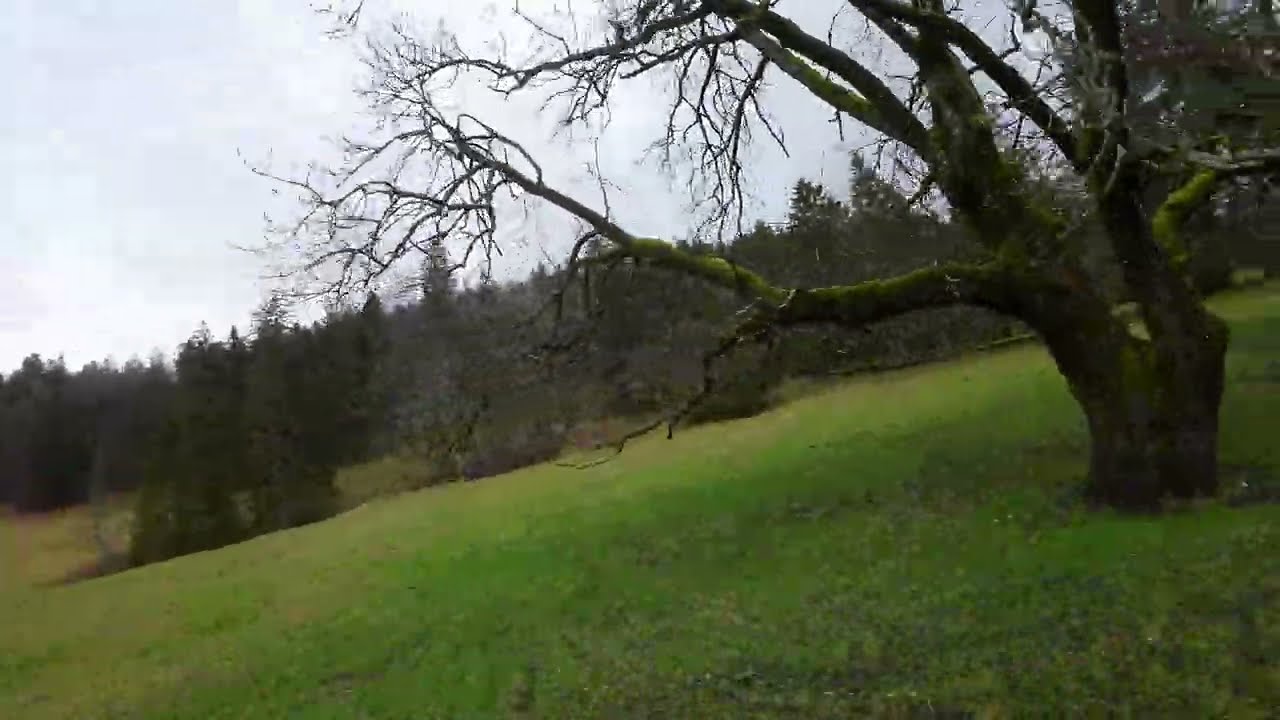This landscape photograph captures a grassy hillside, with the lower part of the slope on the left side of the image and ascending to the right. Dominating the right foreground is a gnarled tree with a wide, stocky trunk and craggy, moss-covered branches that stretch mainly towards the center and top of the image. The tree stands leafless, with its bare branches extending leftward. In the midground on the left side, there are two tall evergreen trees situated between the main tree and the distant horizon. The background features a dense wooded area with a variety of short trees leading up to a tree-lined horizon beneath a clear, light blue sky. The image, although slightly fuzzy, vividly depicts this serene, sloped landscape.